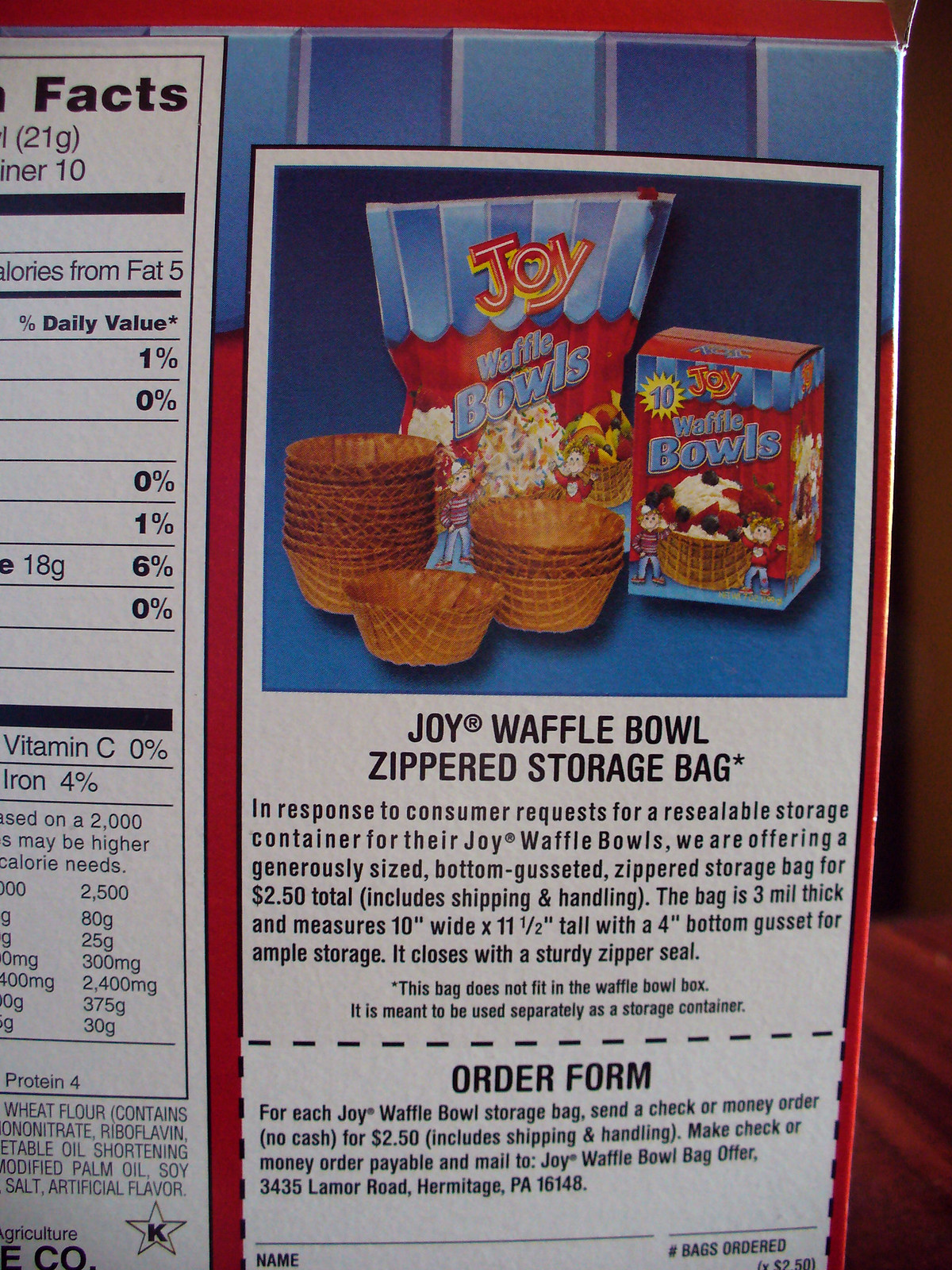This is a color photograph with a vertical rectangular orientation. The image is a close-up of the back of a paper box containing Joy Waffle Bowls, a product where waffle cones are shaped like bowls. The box, printed in vibrant colors, prominently features the brand name "Joy" written in red and yellow, cartoonish letters on a red and light blue design. 

On the right side of the box, partially visible are the nutritional facts and a block of text about a zippered storage bag, next to a small image that also says "Joy Waffle Bowls." The central image on the box depicts a stack of the golden-brown waffle bowls, along with one bowl positioned in front to detail its shape and texture. The scene shows suggestions for serving, such as using the bowls for ice cream, with an illustration demonstrating vanilla ice cream topped with blueberries and strawberries.

In the background on the right, there's a wooden floor and what appears to be a wooden door or wall, adding to the cozy and homely feel of the product display. At the bottom of the box, an order form is partly visible for those interested in purchasing additional zippered storage bags for the waffle bowls.